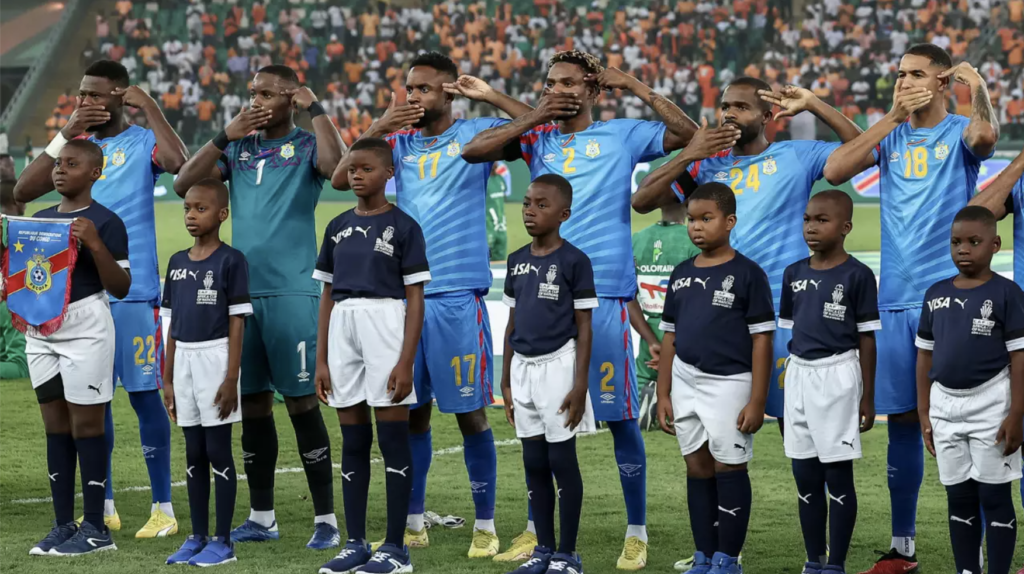The image captures a vibrant daytime scene in a stadium, where a group of six soccer players, dressed in blue jerseys adorned with yellow numbers, stand prominently on a lush green grass field. Among them, one player is distinguishable in a green jersey with a white number. Each player is covering their mouth with their right hand while pointing towards their temples with their left index and middle fingers. Positioned in front of the players is a line of young boys, each clad in a navy blue top and white shorts, resembling a uniform. These boys are holding a flag. Behind the players, the stadium's stands are filled with a diverse crowd, observing the scene intently. The image is bathed in natural lighting, enhancing its clarity and vibrant colors, which together encapsulate the spirited atmosphere of the event.